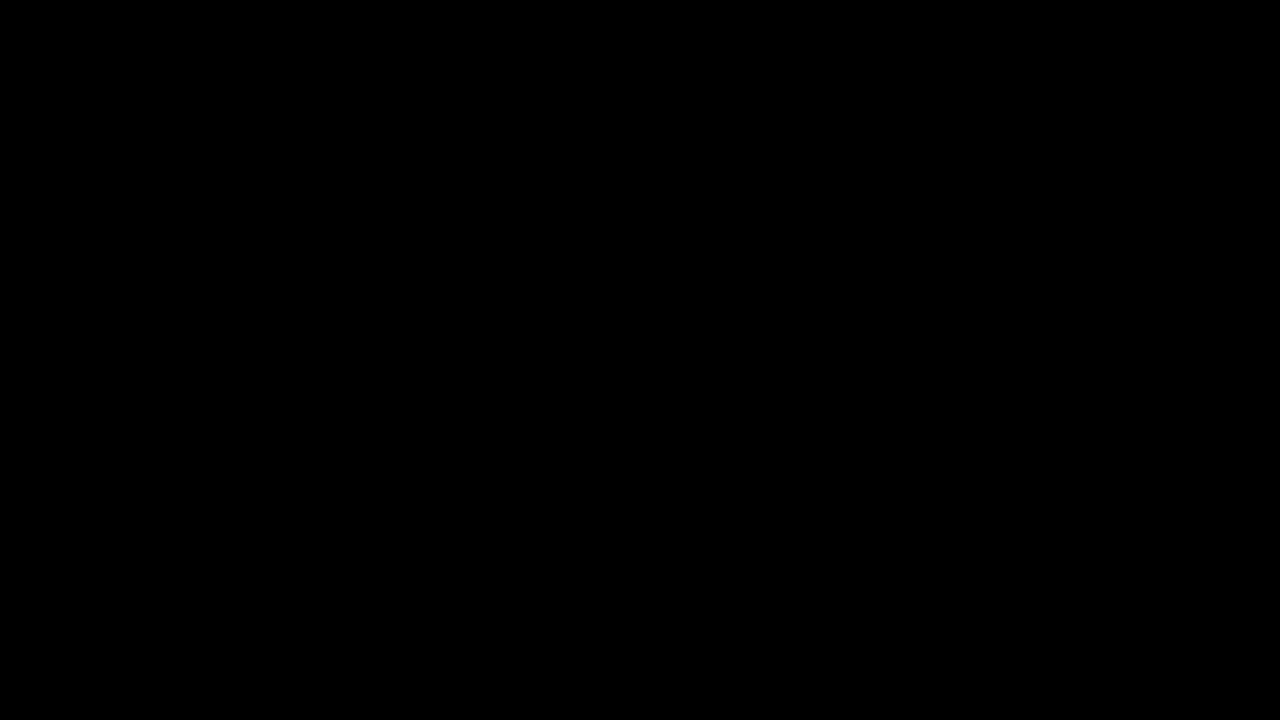The image depicts a completely solid black horizontal rectangle, devoid of any text, images, or objects. The black background fills the entire frame uniformly, with no variations or interruptions in the color. The proportions of the rectangle are notable, with its width being approximately 1.5 times longer than its height. This pure black image offers nothing else to see or interpret, maintaining a consistent and true black color throughout.